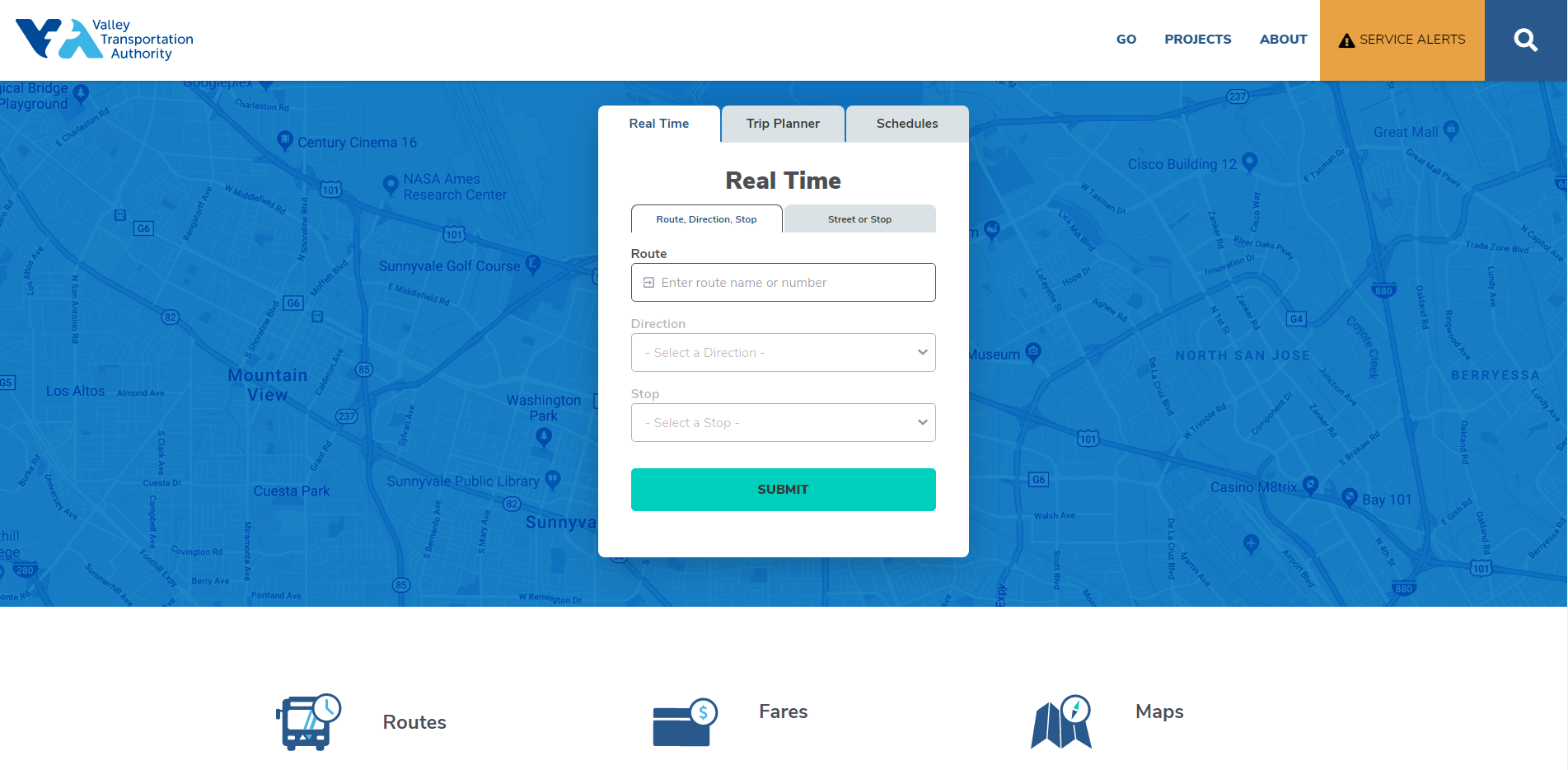The image depicts a complex interface design with various elements and icons. On the left side, there is a logo comprising two stylized letters: a dark blue "V" and a light blue "A". Adjacent to the logo, there are green words, the content of which is unspecified. Further to the right, there are blue words, followed by an orange rectangle containing a triangle pointing upwards and black text. Next to it is a blue square with a magnifying glass icon.

Below these elements, the background shifts to a blue overlay featuring a map, which includes symbolic map points highlighting specific locations. A white rectangle with a white tab at the top, inscribed with words, is present, accompanied by a gray tab with words and another gray tab with a single word. Below this section, the term "real-time" is displayed.

The interface continues with several gray-outlined rectangles, each containing text. These include multiple gray rectangles containing words, interspersed with single words, and a gray rectangle with an arrow pointing downwards, followed by more text. A blue-green rectangle at the bottom features the word "submit."

Underneath this, an image of a blue bus is displayed, labeled "routes." This is followed by a rectangle with a white line and a circle on the right-hand side that includes a number and is labeled "fares." Finally, there is an illustration of a map with a circle containing an indistinct element, labeled "maps."